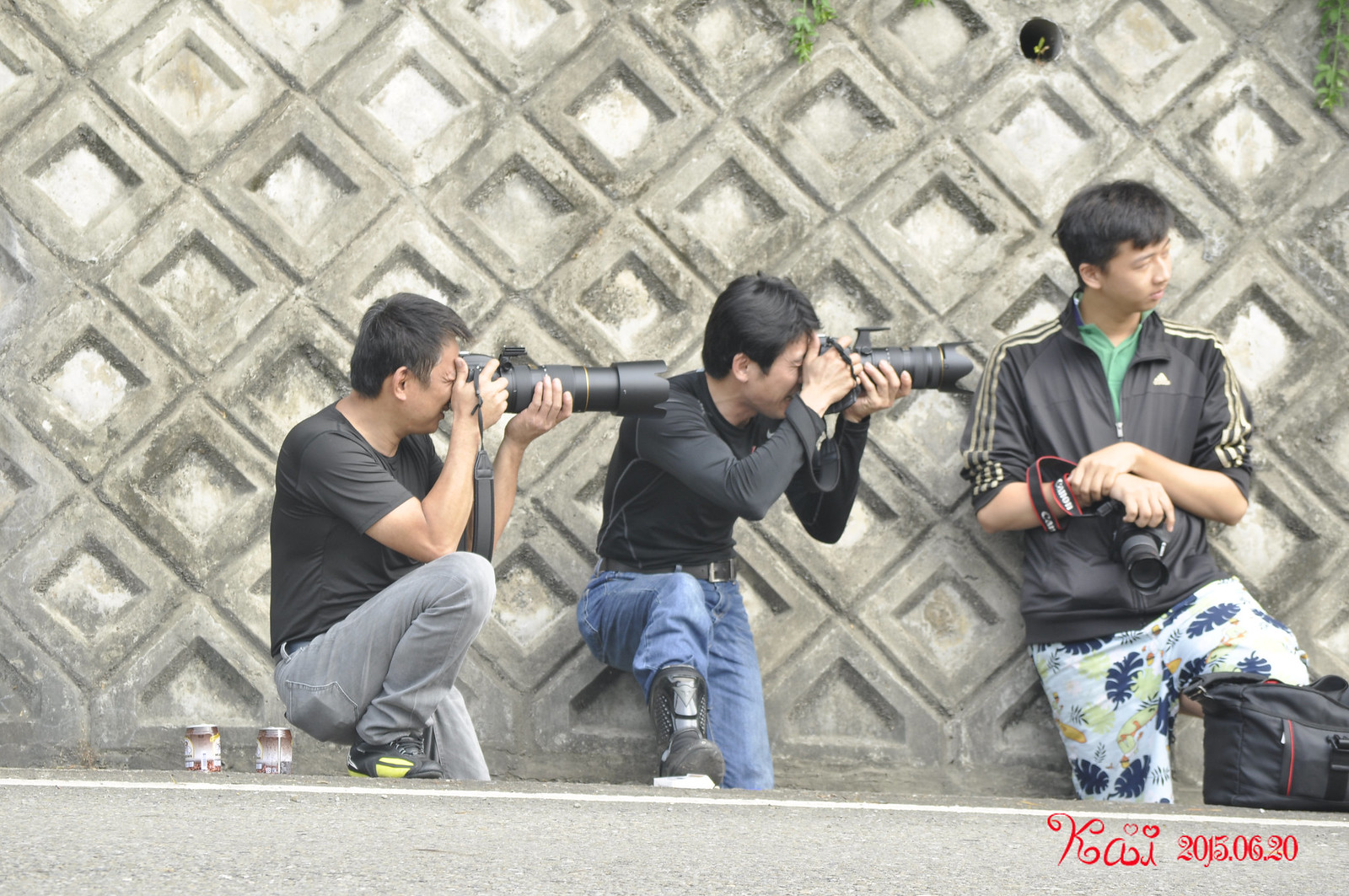In this photograph, we see three Asian photographers standing in front of a distinctive gray concrete wall adorned with a diamond-shaped pattern. Each of the photographers has his foot raised and resting on a shorter concrete divider in front of the wall. The man on the left is dressed in a black shirt and gray pants, holding a black camera with a long lens up to his eyes, aiming to the right. The photographer in the middle is similarly posed, wearing a black shirt and blue pants, also peering through a black camera with a lengthy lens pointed in the same direction. The third man on the right contrasts with his peers by holding his camera down in front of his torso, not actively taking a photo. He is adorned in a black Adidas jacket with gold stripes down the sleeves and light-colored pants decorated with blue, yellow, and orange leaves. At their feet lies a black duffel bag along with what appears to be two jars resting on the concrete wall. Notably, in the corner of the image, the date "KAI 2015-06-20" is elegantly inscribed in red cursive. The trio is set against a gray paved walkway that aligns with the bottom edge of the picture.